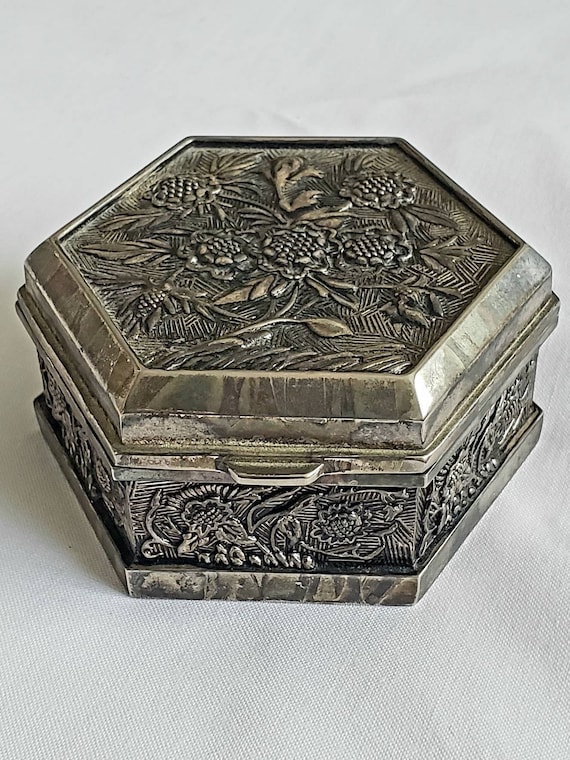The image depicts a hexagonal, weighty box that appears to be made of a tarnished silver or pewter-like metal. The box, which rests on a white cloth background that fades out of focus towards the top, is adorned with intricate engravings of a floral pattern that may include leaves and pine cones. The design elements are raised, giving a three-dimensional texture to the surface. The lid, which is slightly more tarnished with hints of beige and black, covers a matching bottom portion that appears somewhat cleaner and darker. The box is closed, preventing a view of its interior.